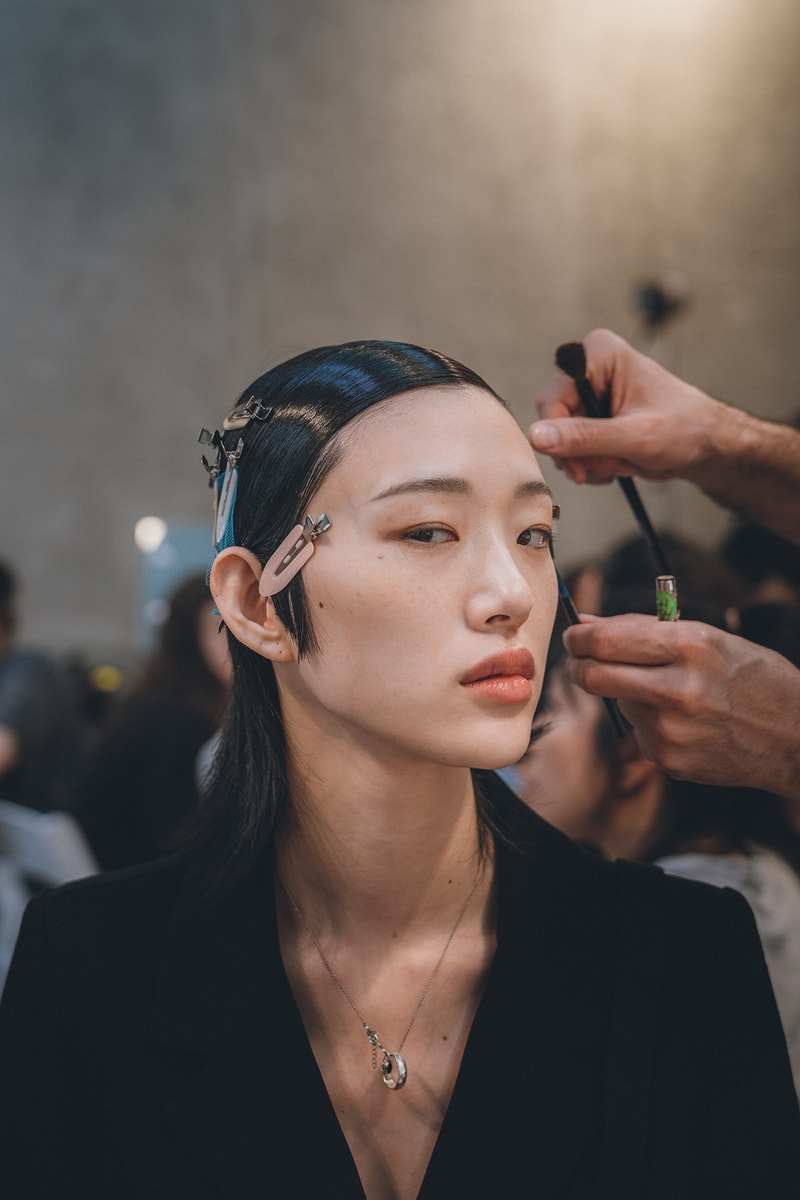The image features a young East Asian woman, likely a model, captured from the chest up. She possesses a striking androgynous appearance, with straight eyebrows, full lips of a vibrant peach-pink hue, and sleek, shiny, straight black hair that is clipped back with various barrettes, including noticeable pink and blue ones on the left side. Her head tilts slightly to the right as she directs a serious, sideward glance to her left. The woman is dressed in a structured black blazer with a deep V-cut, exposing a delicate chain necklace with a plain silvery band hanging from it. 

In the foreground, a pair of hands, presumably those of a hairstylist or makeup artist, emerges from the right. The right hand holds a black makeup brush, while the left hand seems to be adjusting her hair. The background is softly blurred, featuring hints of another female figure with dark hair, likely engaged in similar grooming activities, all set against a light reddish backdrop. The overall composition suggests a setting related to fashion or hairdressing, where the model is being prepped, highlighting her poised and attractive profile amidst an atmosphere of meticulous styling.